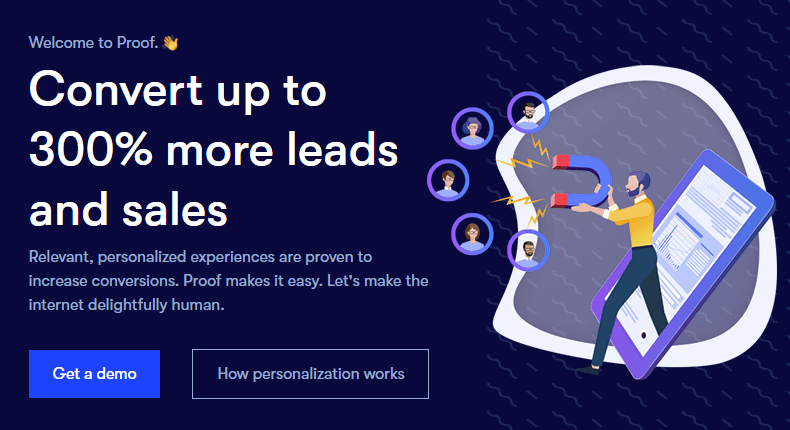In the top left corner of this image, the words "Welcome to Proof." are displayed, followed by a waving yellow hand emoji. Centered below this text, in larger white font, are the words "Convert up to 300% more leads and sales." Directly beneath this, smaller text reads, "Relevant, personalized experiences are proven to increase conversions. Proof makes it easy. Let's make the Internet delightfully human."

In the bottom left corner, a blue box features the text "Get a Demo" in white. Adjacent to it on the right is a larger box, matching the dark blue background of the entire image, with the text "How Personalization Works."

On the right side of the image, a man emerges from an iPad, holding a large magnet pointed at five floating bubbles, each containing an image of a person. The man sports a black beard, short black hair, a yellow shirt, blue pants, and black shoes.